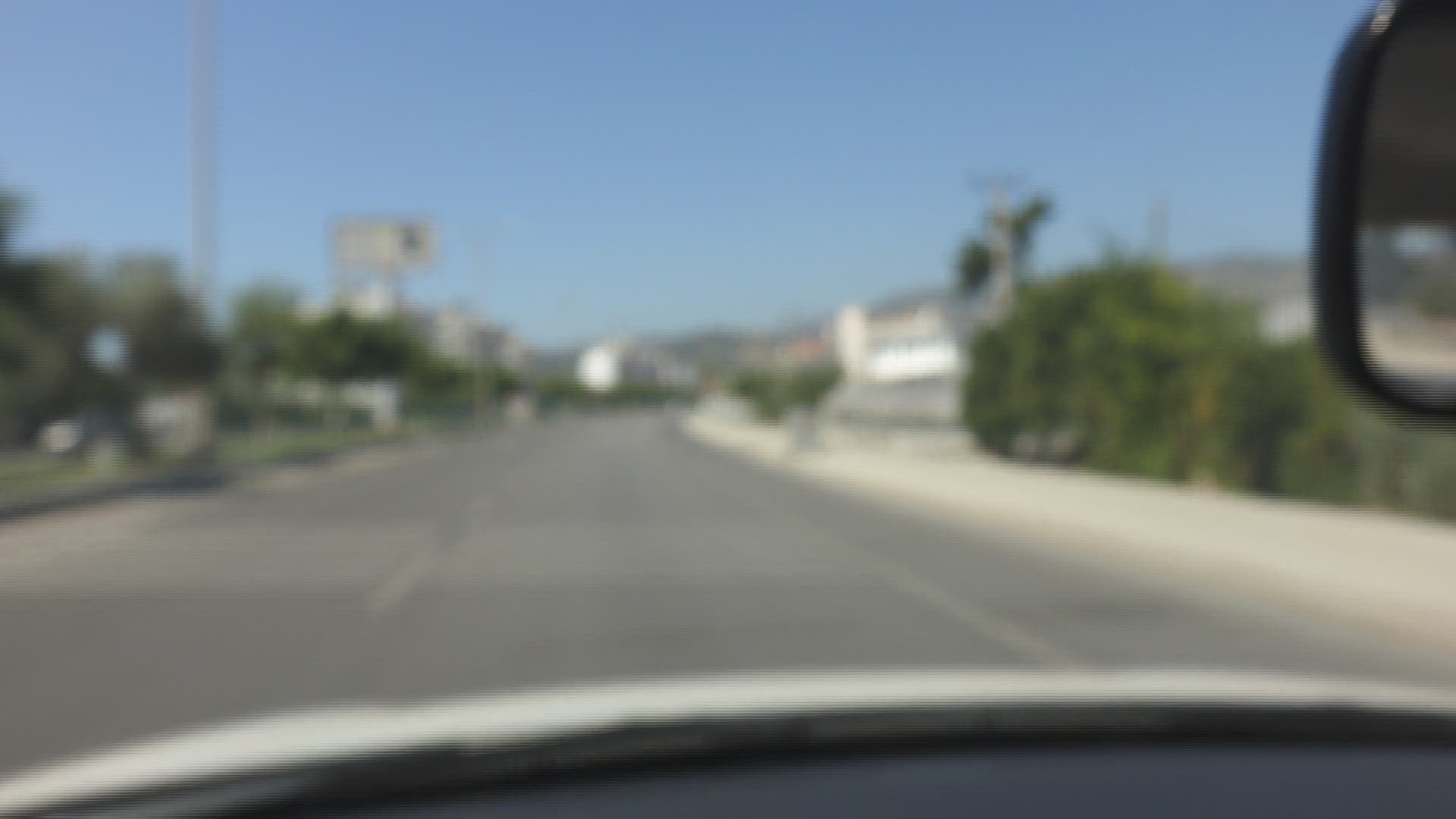Through the slightly blurred truck window with its gray door and black side mirror, a scenic vista unfolds. The view extends to a paved road bordered by a sidewalk that stretches into the distance, interspersed with small trees and bushes. In the background, a cluster of buildings punctuates the horizon under a clear blue sky. Dominating the scene is a tall silver pole, flanked by street signs and light poles, extending the urban landscape into the far distance.